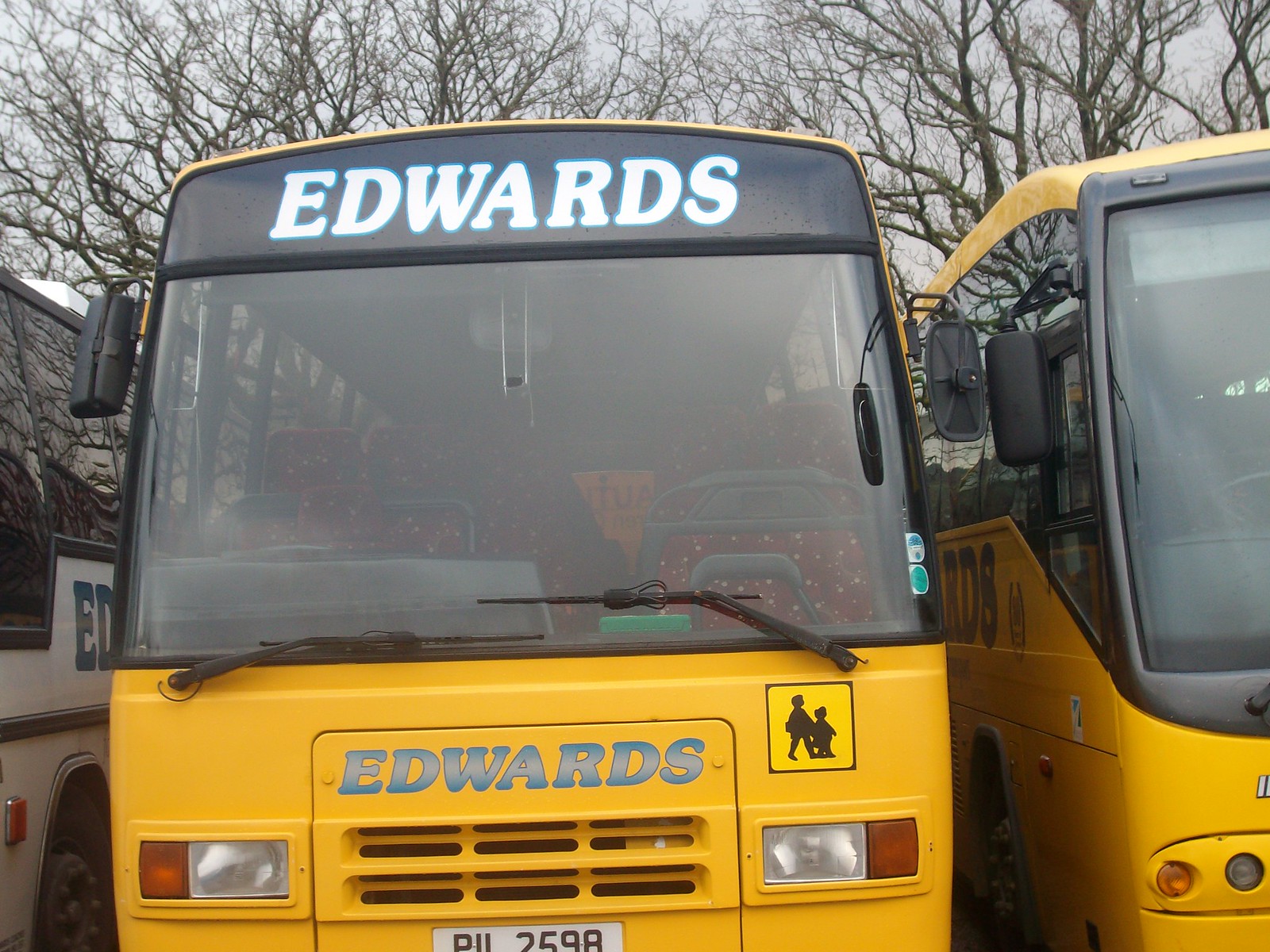In this outdoor photograph, three buses are prominently visible under a gray sky, with a backdrop of leafless trees indicating a fall or winter setting. At the center stands the focal bus, a large yellow vehicle with a boxy front. It features a black strip at the top with the name "Edwards" in white lettering outlined in blue. Below, the front of the bus also displays "Edwards" in silver lettering. The bus has a vast, rectangular windshield, clear rectangular headlights on the left and right, and orange turn signals beside them. A white license plate is positioned below the front grill. To the right of the center bus is another yellow bus, while to the left, a white bus is parked. The scene includes a safety symbol—a yellow square with a silhouette of an adult and child—emphasizing the buses’ role as school transportation. The entire scene is devoid of passengers and evokes an empty, almost serene atmosphere.